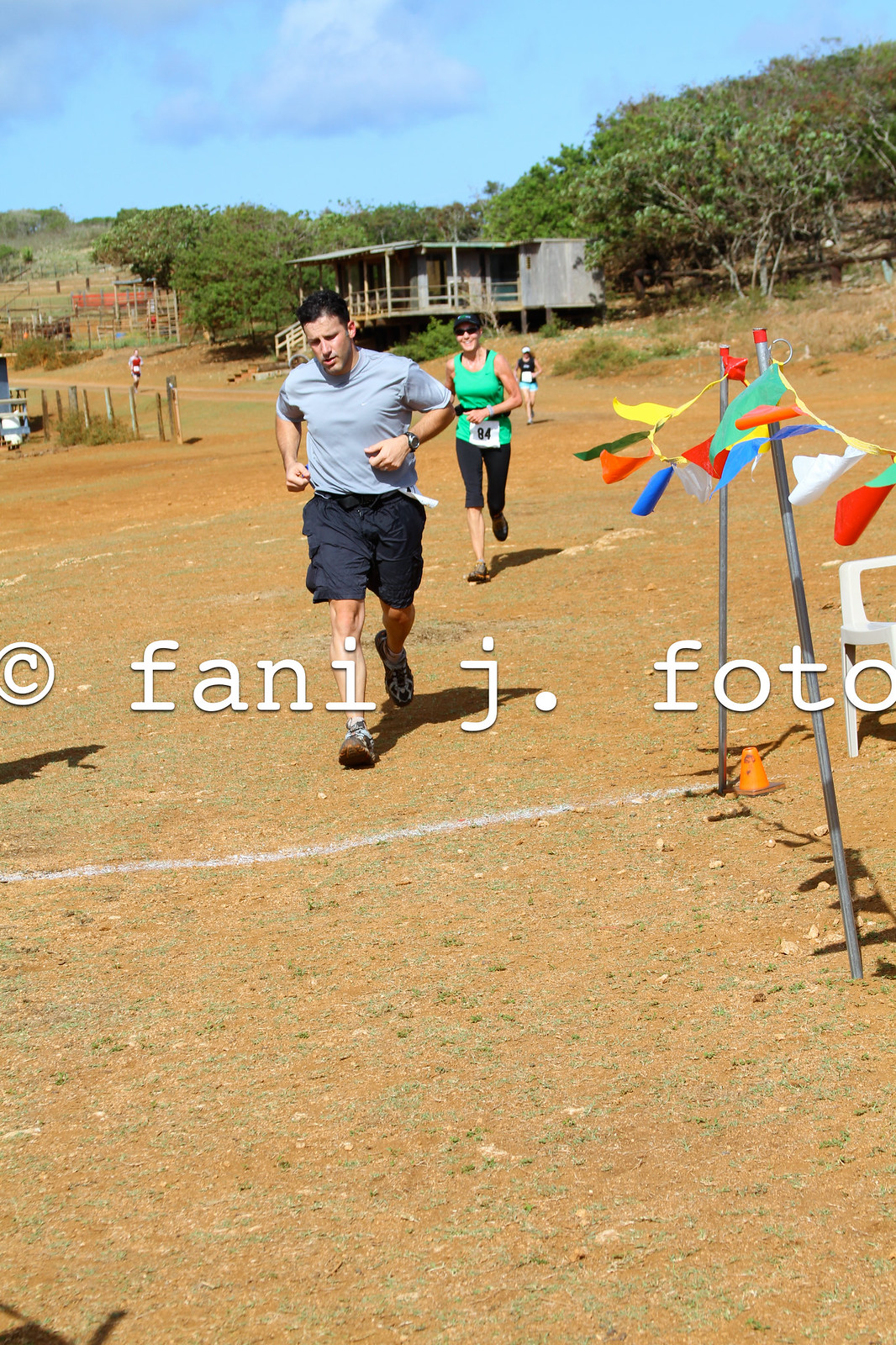In this outdoor photograph, the background showcases a blue sky above a green tree line interspersed with rough wooden buildings that resemble shacks, highlighting a rustic setting. The foreground features a dirt path where several people are running, hinting at a race environment marked by a white line and an orange cone that likely signifies a finish line or starting point. Dominating the scene is a man in a light blue top and dark blue cargo shorts, caught mid-jog as he nears the white line. His right foot extends forward, indicating his slow but steady pace. 

Close behind him, a woman is also jogging, wearing a green tank top, black capri-length leggings, and a hat. Ahead of these two central figures are more runners, including a smaller, less distinguishable individual dressed in dark clothing with green shorts. Two metal poles adorned with multicolored pennant banners—red, yellow, blue, white, and possibly green—stand to the right side of the path, adding a festive touch to the scene. 

Stamped prominently across the middle of the image is a watermark that reads "FANIJ.FOTO," indicating the photograph's copyright. The overall terrain appears dry and gravelly, adding to the desolate, desert-like atmosphere of the race setting.